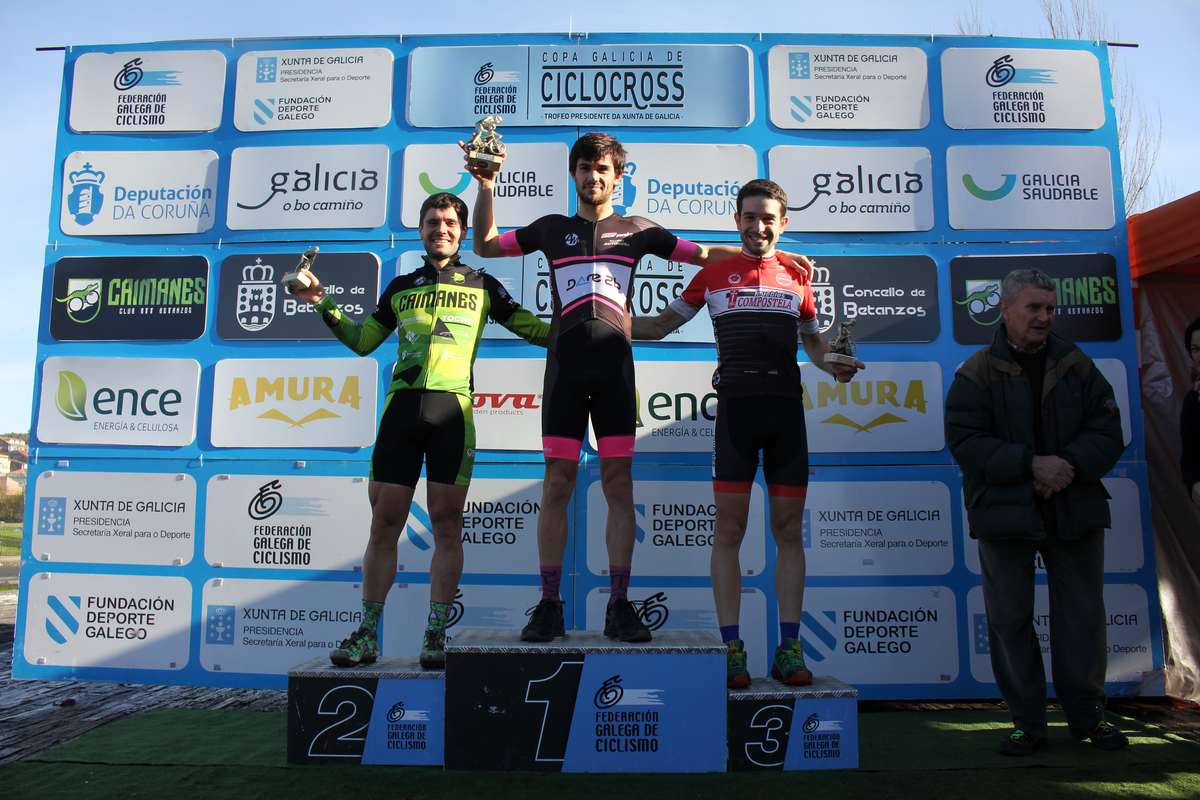The image shows three young male cyclists in their early 20s standing on a podium, celebrating their victories in a cycling competition. They are positioned on painted platforms of varying heights, signifying first, second, and third places, and are holding trophies. The winner, centered on the tallest podium, proudly displays a gold bicycle trophy. He is dressed in a black and hot pink cycling uniform with black shorts and shoes. To the left on the second place podium, the cyclist wears a black and lime green jersey and holds a similar trophy. The third place cyclist, on the right, sports a red jersey with a white stripe, black pants, and green shoes. Behind them, a large banner filled with various sponsor logos, including prominent names like "Cyclocross," "Entz," and "Amira," stretches across the frame. The scene is set on grassy ground, with an additional man in a warm jacket and black pants standing to the side, observing with his hands clasped.